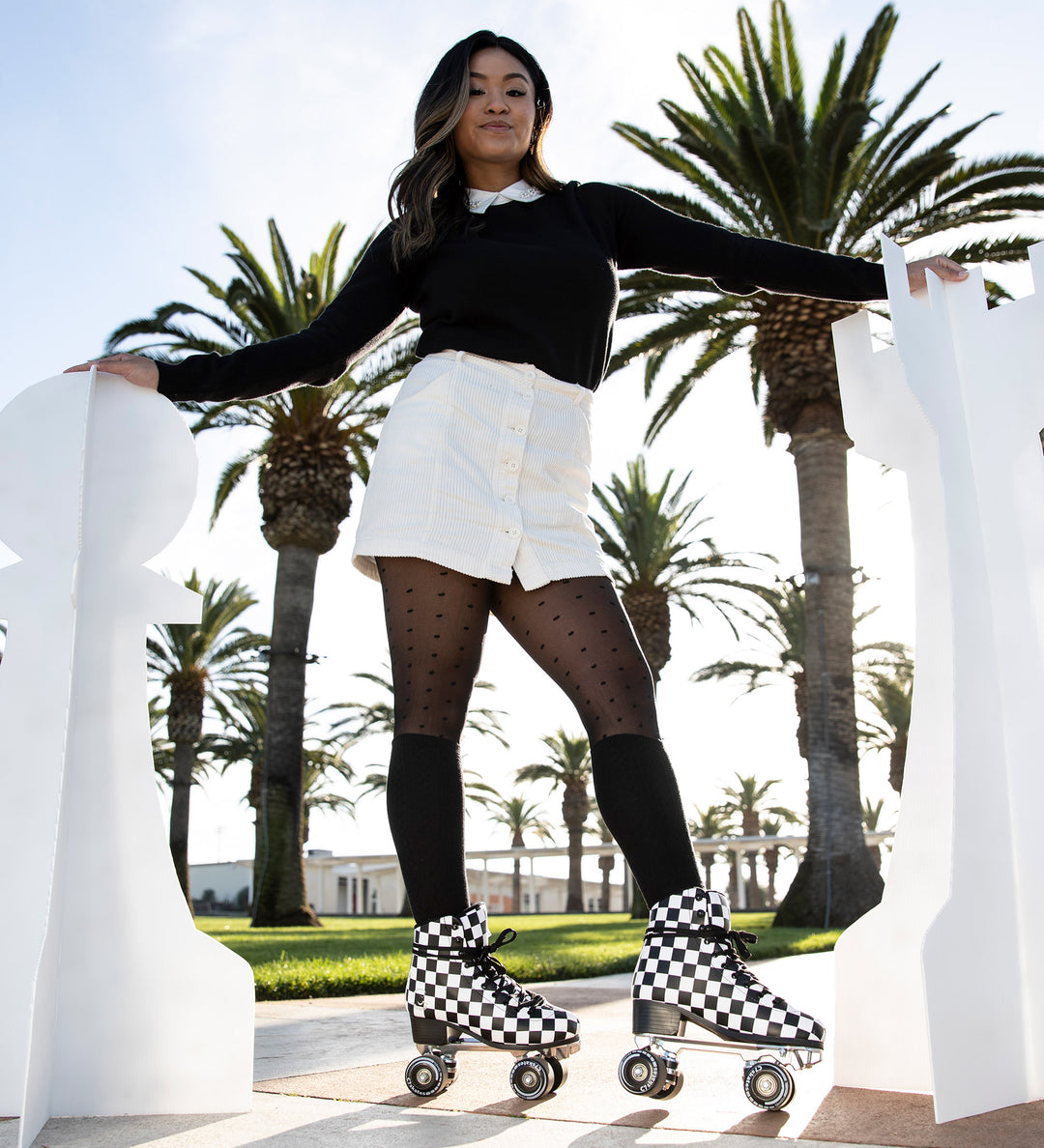The image is a color photograph of a young Asian woman, possibly an older teenager, in a confident power stance. She has dark brown hair with hues of black, and she is wearing a black top layered over a white collared shirt. Her bottom attire is a bit ambiguous—it could be white shorts or a white skirt—and she pairs it with black leggings adorned with black dots and long black socks. On her feet, she sports black and white checkered roller skates. The scene is set in a tropical location, evidenced by the abundance of green palm trees with brown trunks in the background. The sky is a light shade of blue. The setting includes a tiled path and what appears to be a life-size chessboard with visible chess pieces like a rook and a pawn. The woman stands on concrete, and she seems quite pleased, adding a sense of lightheartedness to the bright, sunny day.